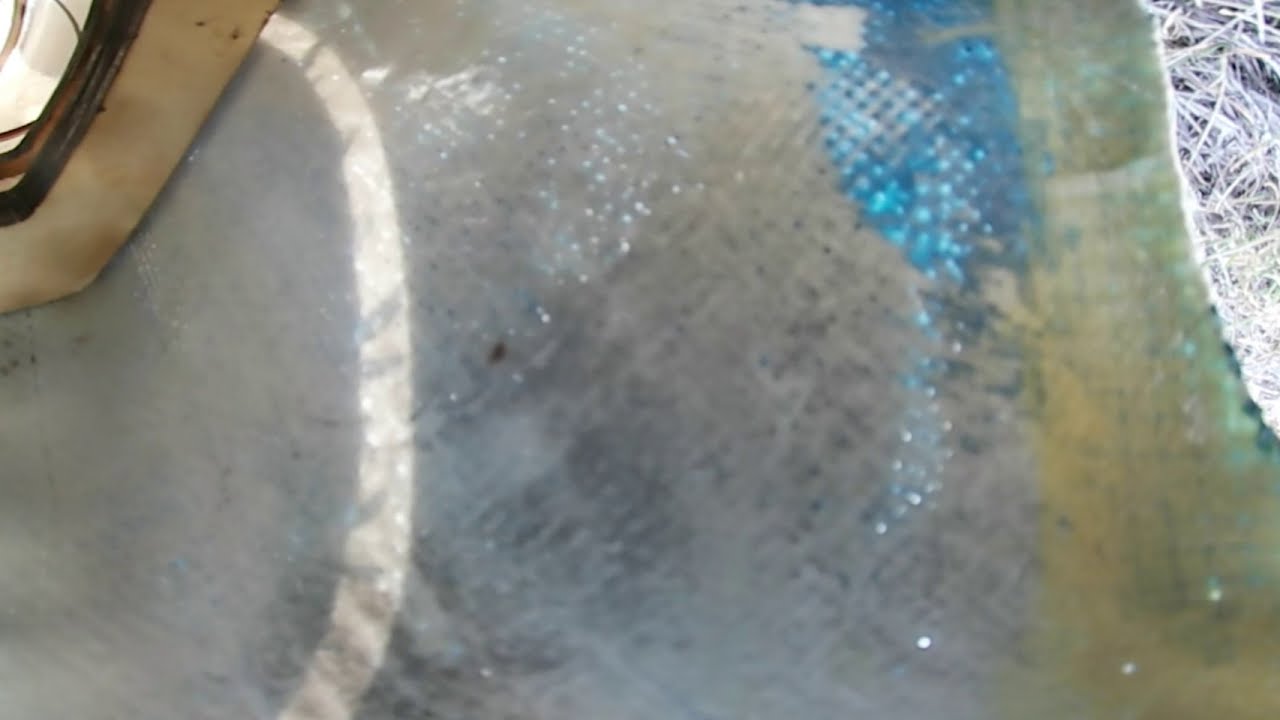The image depicts a rectangular mat lying on the ground, surrounded by dried grass on the right edge. The mat is extremely dirty and features a variety of stains and discolorations. The left side of the mat has a prominent speckled white patch, while the right side boasts a solid blue spot. The mat’s colors range from gray to white, speckled to darker gray, transitioning into blue, a brighter blue, yellowish, and faded green hues. The surface of the mat appears grainy and weathered. Additionally, in the top left corner of the image, there is a glimpse of a car’s tan-colored fender and headlight, with sunlight casting a rounded strip of light across the mat.